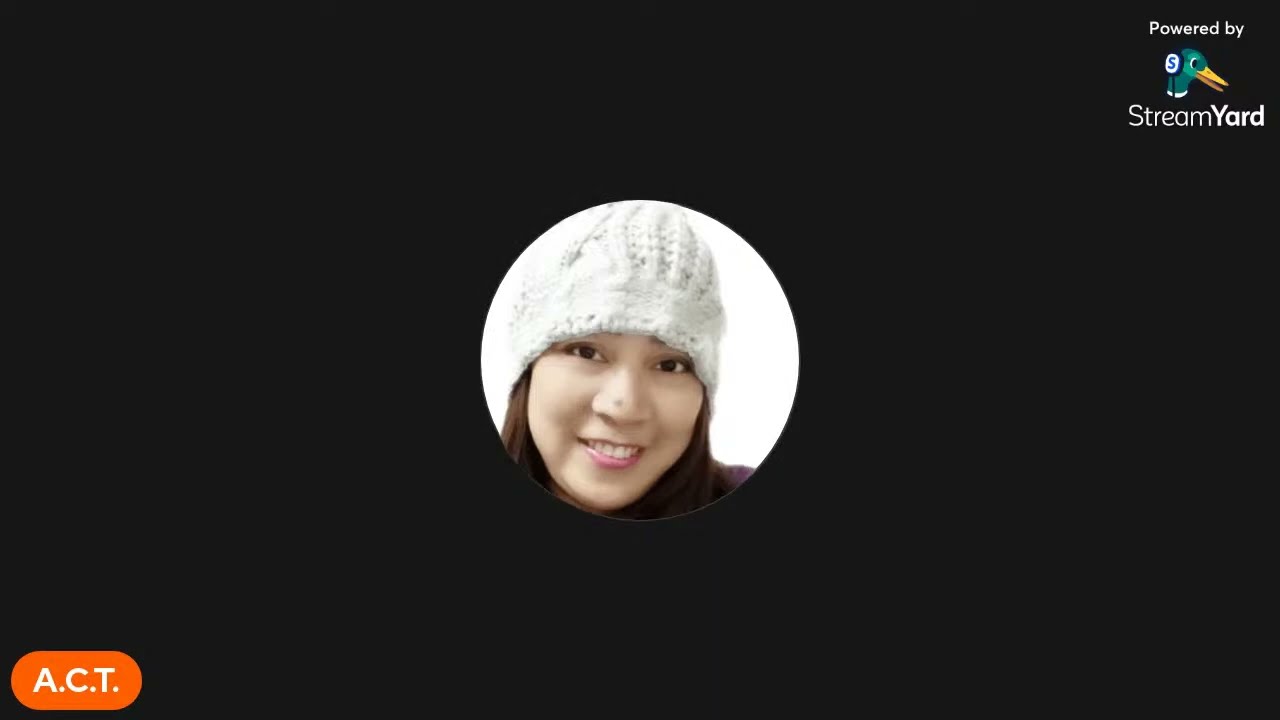In the center of a black rectangular image with a glittery finish, a young woman, possibly Asian, is featured inside a circular thumbnail. She has dark brown hair and is wearing a white knitted skullcap. Her face, highlighted by a white background, shows a cheerful smile, revealing her upper teeth, and she may have a small nose piercing. She is wearing pinkish lipstick. The upper right corner of the image displays white text reading "Powered by Stream Yard," with a duck's head logo bearing the letter "S" in between "Powered by" and "Stream Yard." In the lower left corner, an orange oval laid on its side contains the text "A.C.T." in white capital letters.